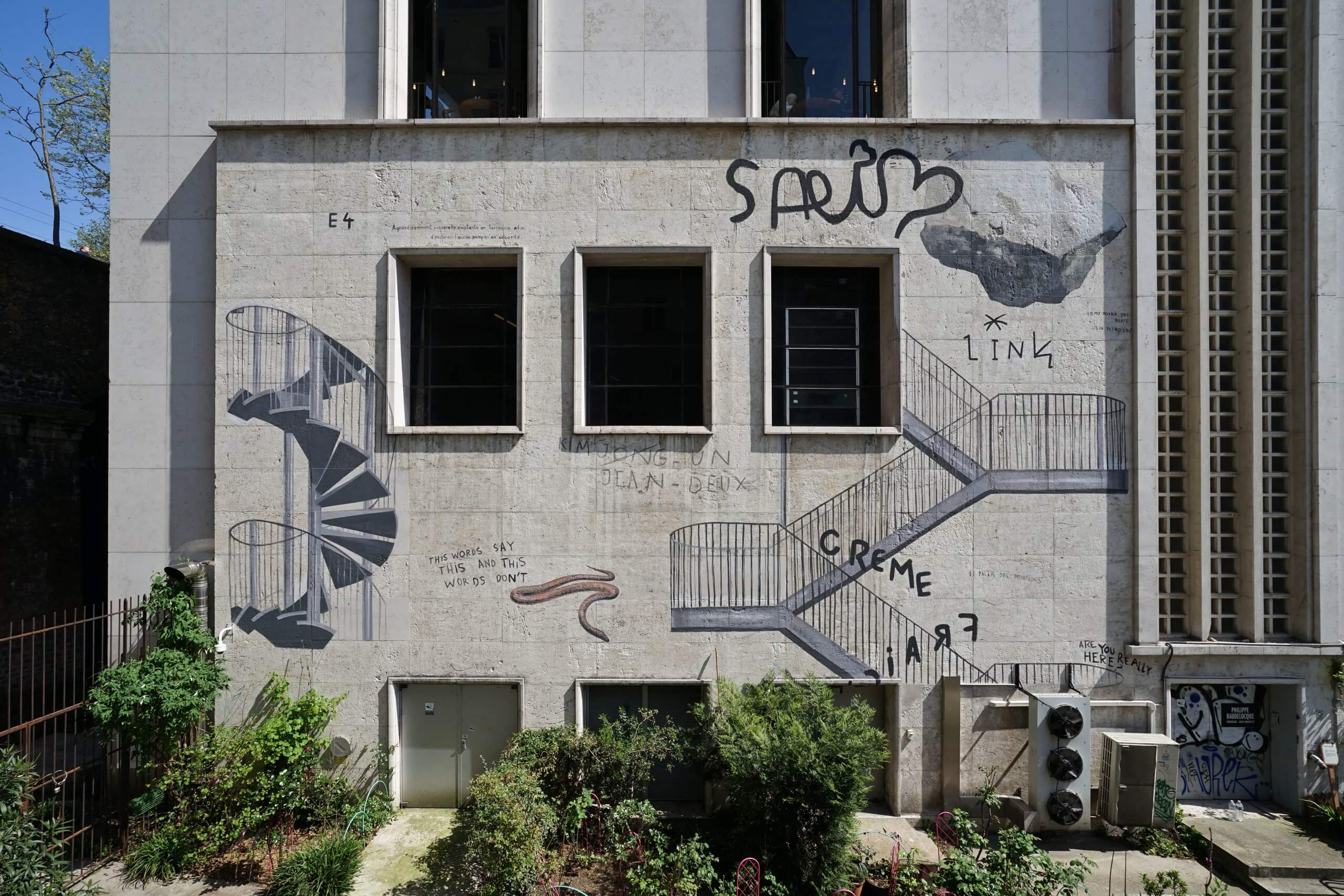This daytime photograph showcases a multi-story gray concrete building with large, rectangular windows that extend into darkness. The main focus is on the side of the building, adorned with various pieces of graffiti art. Notably, there are two painted staircases: a gray spiral staircase on the left, and a classical staircase on the right that ascends in segments, leading to a second-story window. Above the classical staircase, a large painted boulder appears poised to fall. Additional graffiti includes black lettering spelling "CREME" and "F-R-A-I-C," the latter written at an angle, descending from the top right to the bottom left. The top portion of the building features more text and heart shapes. At the base of the building, green bushes add a touch of nature. The image captures both the main structure and parts of adjacent building segments, with some industrial equipment like an electrical panel and an AXE unit visible in the corner. The sky in the top left is a clear blue, free from clouds.